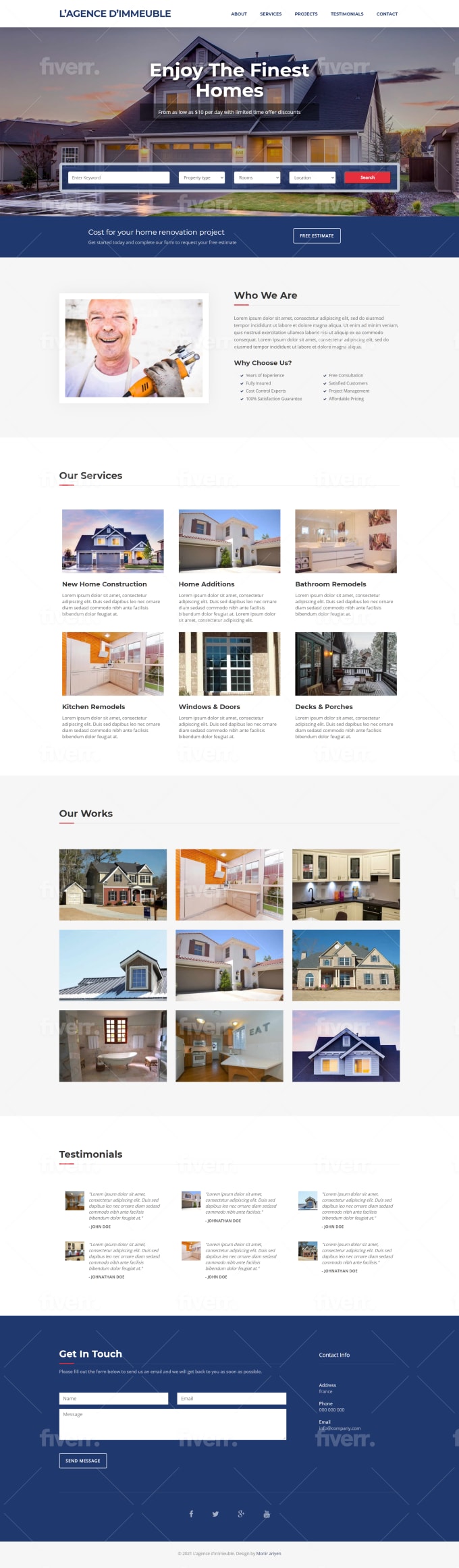A lengthy, single-image web page is depicted, making it challenging to read due to its compressed format. At the top of the page, the title is in French, "Légence Communable" (or something similar), accompanied by a banner that reads "Enjoy the Finest Homes." The banner features an image of a two-story suburban house and has a visible Fiverr watermark, suggesting that the image was crafted by a freelancer but the watermark wasn't removed.

Below the banner, there's a section where users can enter an address, as well as details like "beds" and "baths." Scrolling down reveals a somewhat eerie stock photo of a man holding an ambiguous tool. Further down, the section labeled "Our Services" includes additional images of houses, alongside text that is largely unreadable. One subsection, "Our Works," shows more photos of modern, suburban homes, many featuring gabled roofs. The page concludes with a "Get in Touch" section at the bottom.